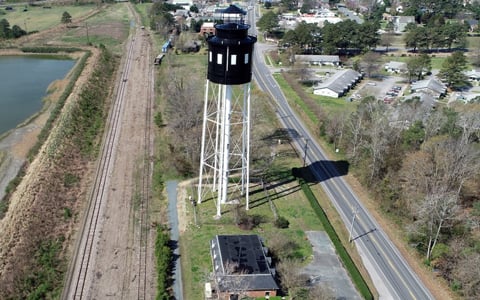The photograph is an aerial view of a rural town's landscape, featuring a predominating black and white water tower. The tower stands on white poles with a black tank, decorated with white squares, creating a distinctive pattern. The top of the tank, which might be mistaken for a lighthouse due to its windows, suggests it could be a lookout or guard tower. To the left of the tower, there is a rectangular, man-made reservoir bordered by both dead and flourishing vegetation. Adjacent to the reservoir are train tracks, a small dirt road, and further to the left, a mix of brown ground and additional bodies of water. In the foreground, there's a small brick house with a green roof. On the right side of the tower, a two-lane paved road stretches into the background, leading to a distant town. The photograph, seemingly taken from a plane or drone, captures the tops of buildings and trees, casting long shadows, indicating a bright sunny day, likely in late fall or winter as most trees are bare.